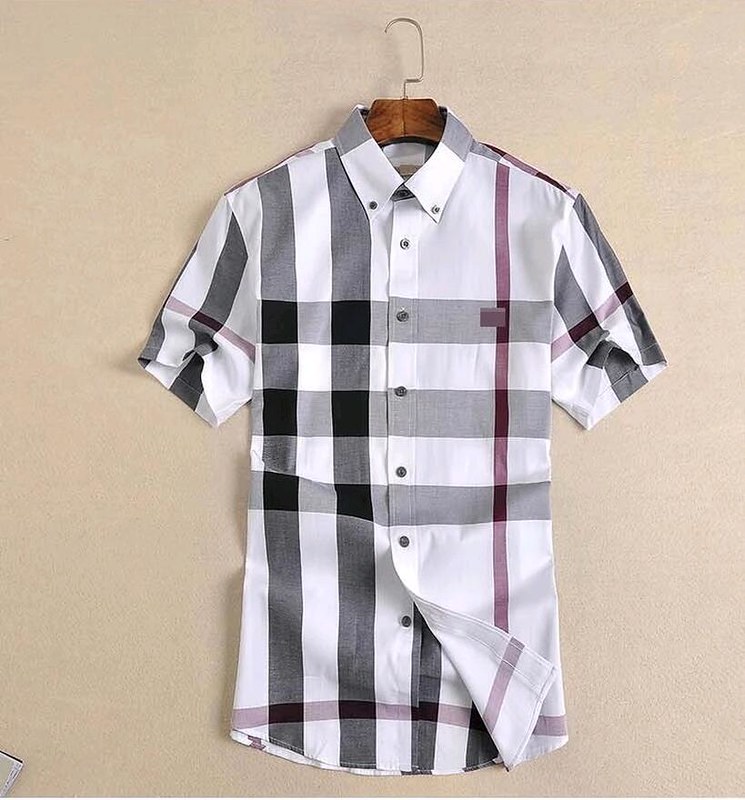This photograph features a men's short-sleeved button-up shirt displayed on a wooden hanger with a metal hook. The shirt is set against a tan background, lying flat with one corner slightly folded. It has a striking design of vertical and horizontal stripes in black, white, gray, and red. Six black buttons run down the front, with the bottom button unfastened. The collar is secured by two buttons. The vertical black and thin red stripes contrast sharply with the gray ones that traverse the chest. A small label is visible on the chest. Additionally, light rose and red lines are noted at various points, including over the sleeves and near the shirt's bottom edge, adding a touch of color to the checkered design. The hanger, with its golden-colored wire, complements the dark wooden hook, enhancing the overall presentation of the shirt.